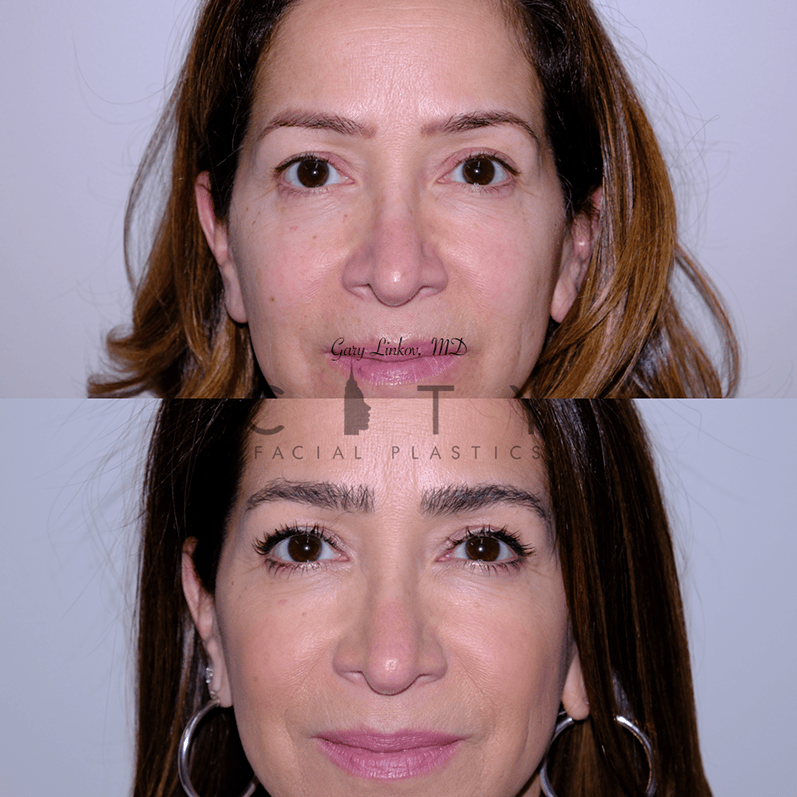In this image, two horizontally aligned photographs, one above the other, depict a woman's face in a before-and-after transformation. Both photos focus on her middle facial area, excluding her chin and the top of her head, set against a grey background.

In the upper photograph, the woman has medium brown hair that lightly frames her face, brown eyebrows, and brown eyes. She is wearing pink lipstick and looks directly at the viewer with a neutral expression. Text overlaid on her lips reads "Gary Linkov MD" in black.

The lower photograph shows notable changes: her hair is now darker, her eyebrows have turned black, and she has longer eyelashes. She is wearing large silver hoop earrings and has a subtle, more youthful appearance with a slight smile. Over her forehead, text reads "Facial Plastics" in all caps brown letters, accompanied by a logo spelling out "CITY" with an outline of a face. The differences emphasize the makeover's impact, particularly around the eyes, hair, and overall expression.